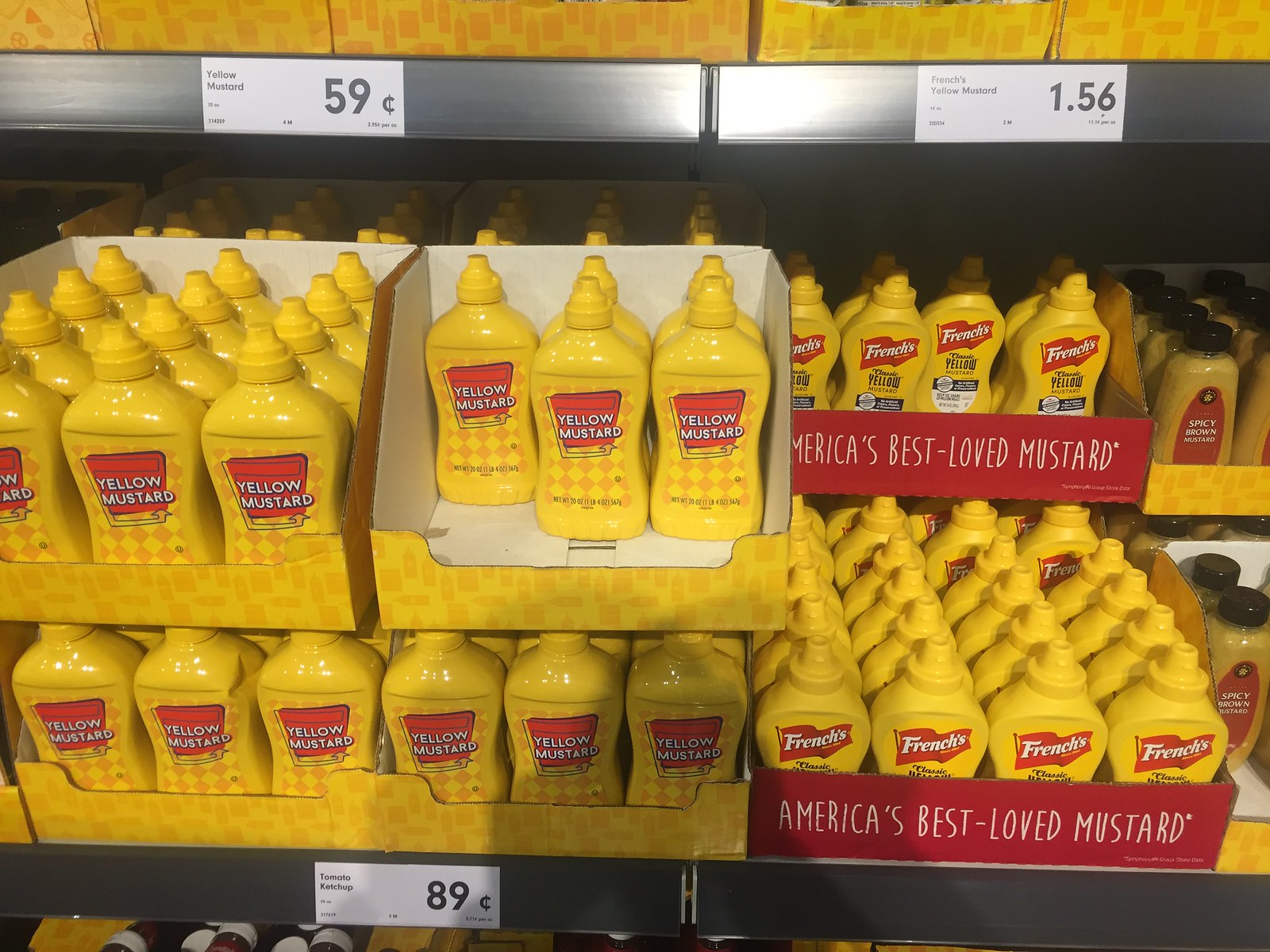The image captures a detailed view of a mustard display at what appears to be a wholesale or grocery store. The camera angle suggests the photographer was standing and looking slightly downward at the shelf. The display features various types of mustard arranged in their original packaging boxes. 

To the left, there are multiple cartons of generic yellow mustard. Each yellow mustard bottle is in a plastic squeeze bottle with a top that features a spout. The top shelf has a price tag indicating 59 cents, while the bottom shelf shows an 89 cents tag, which seems to be mislabeled as it mentions tomato ketchup. This suggests that customers need to look at the tags above the products for accurate pricing.

Adjacent to the generic mustard, there are boxes of French's yellow mustard, recognizable by their red cardboard packaging that proudly claims to contain "America's Best Loved Mustard." The price for French's mustard is marked at $1.56 on the white tags above. The visible quantity indicates that the store might have sold several bottles already, as some boxes appear partially empty.

To the right of French's mustard, another variety, possibly spicy brown mustard, is placed, though specific pricing information for this type is not visible in the image. Overall, the display suggests individual purchase options, emphasized by the pricing tags directly above the products.